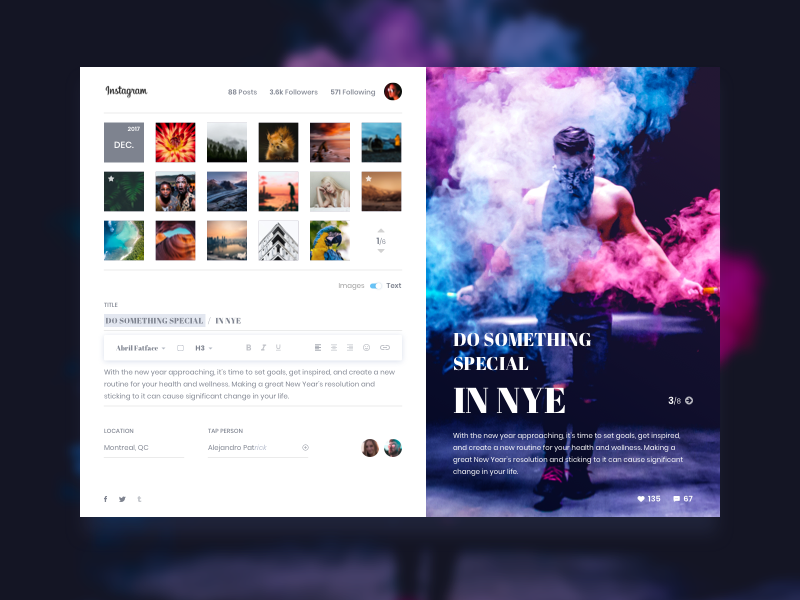In this image, we see an advertisement for Instagram that prominently features a dual-layered visual. The foreground showcases a captivating photo of a shirtless man in a dimly-lit room, with his face partially obscured by a handkerchief. He is holding two colorful smoke sticks - one emitting purple smoke and the other blue - while seemingly in motion. This image is overlaid with text that reads: "Do something special in NYE. With New Year approaching, it's time to set goals, get inspired, and create a new routine for your health and wellness. Making a great New Year's resolution and sticking to it can cause significant change in your life." 

The same striking image of the man appears in the background, adding depth to the visual presentation. The overlay displays social media metrics: 135 hearts and 67 comments, suggesting significant engagement with the post. 

To the left of the main image, there is detailed account information indicating this is an Instagram profile: 88 posts, 3.6 million followers, and 571 following. Various icons and elements provide navigational options within the app. The overall composition effectively promotes the user's Instagram account while encouraging viewers to embrace meaningful New Year's resolutions.